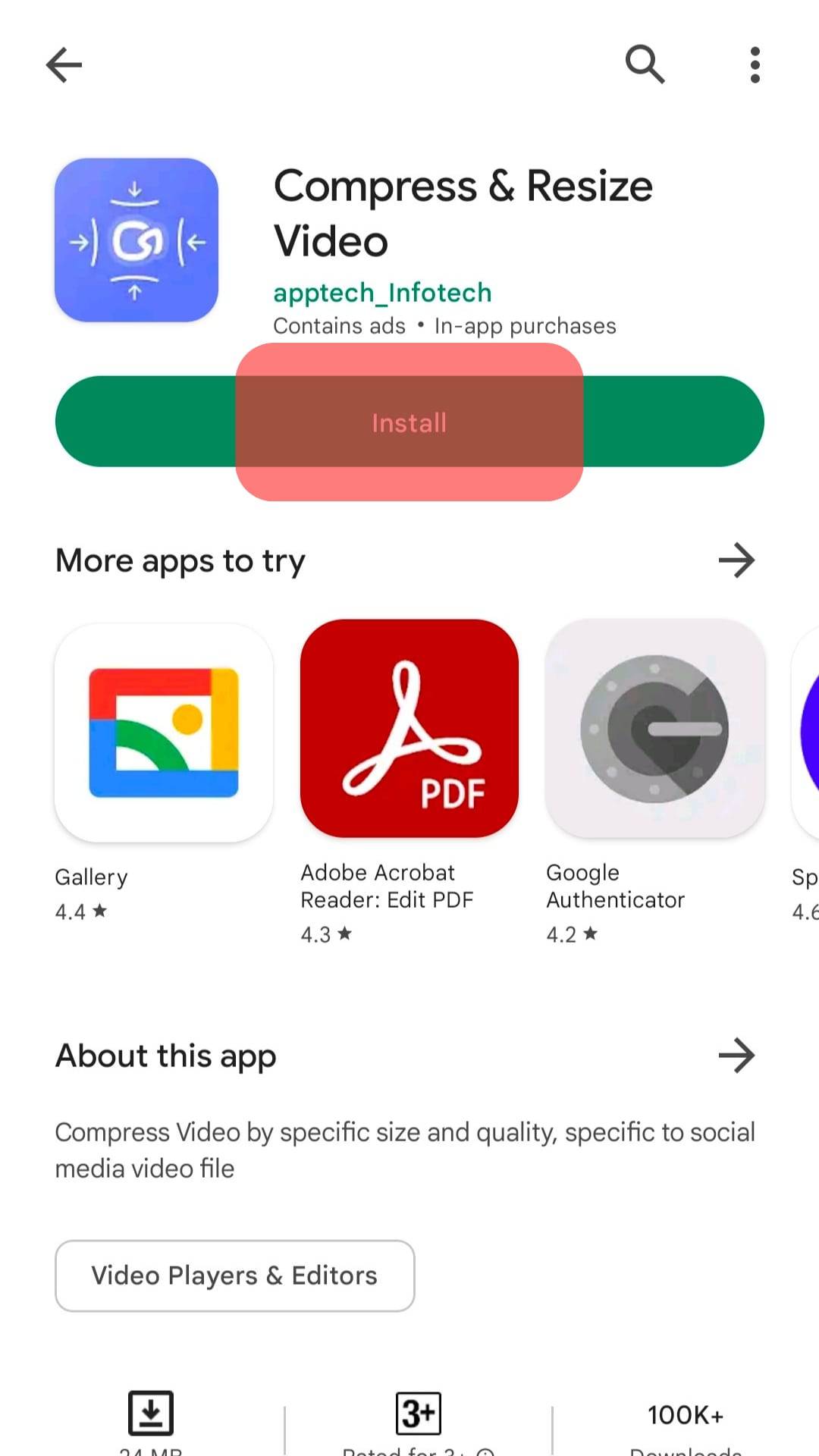Here is a refined and descriptive caption:

---

The screenshot, set against a white background, showcases a detailed interface of a mobile app listing. To the left, an arrow icon and a magnifying glass are visible, followed by three vertical dots representing additional options. The main highlighted app, labeled "aptech_infotech" in green, is described as a compressed and resized video tool that supports ads and in-app purchases. Adjacent to this, a green oval button displays the word "Install" in white, overlaid by a hollow red rectangle. Below, a navigation prompt states "More apps to try," accompanied by a rightward-pointing arrow. 

The screenshot also features a gallery of recommended apps: 
- Adobe Acrobat Reader, Edit PDF (4.3 stars)
- Google Authenticator (4.2 stars)

Each of these recommended apps has a rating clearly displayed beneath them. Additionally, under the "About this app" section, which also includes a rightward-pointing arrow, the description elaborates on the app's functionality for compressing video by specific size and quality tailored to social media platforms. It is categorized under "Video Players and Editors," as indicated within a rectangular label.

---

This cleaned-up caption provides a comprehensive and detailed overview of the screenshot, clearly describing the layout, elements, and functionalities displayed.